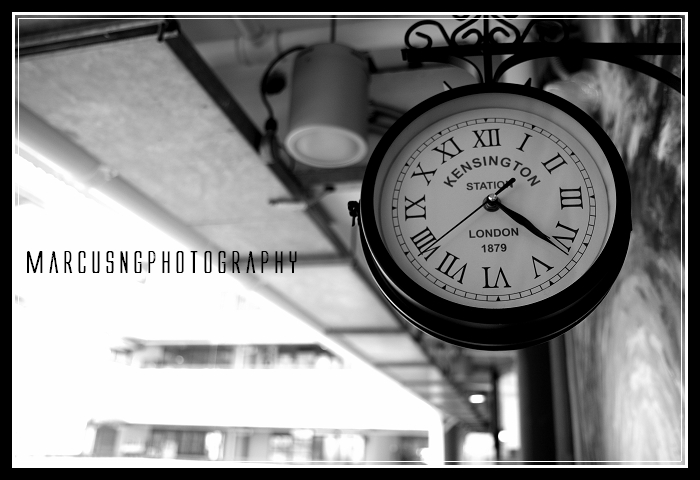This black-and-white photograph is a professional image stamped with the text "Marcus Ing Photography" horizontally across the middle from the left-hand side. The focal point of the photograph is a classic, metal, black clock mounted on a wrought iron arm extending from a wall on the right. The clock features Roman numerals and a white face with the words "Kensington Station" prominently displayed, indicating its historical importance as a station in Kensington, London, established in 1879. Beneath the clock, there is a covered platform area, with bright sunlight sweeping in from the left, creating an overexposed and whited-out background. Blurred out buildings and details such as a cylindrical recessed light above, suggest an outdoor railway station setting, enhancing the timeless and nostalgic atmosphere captured by the photographer.